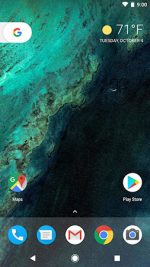This is a blurry screenshot of an Android smartphone's main home screen. The background wallpaper features an oceanic theme with shades of dark green, resembling resin or marble variations. At the bottom of the screen, above the home button, are five app icons: Phone, Messages, Gmail, Google Chrome, and Camera. Above these, a small upward-pointing arrow indicates that more apps can be accessed by scrolling. The Play Store app is positioned on the right-hand side, while Maps is on the left. Towards the top of the screen, the weather widget displays a temperature of 71 degrees Fahrenheit on the right, with the Google Search bar located on the left. In the top right corner, indicators for battery percentage and time are visible.